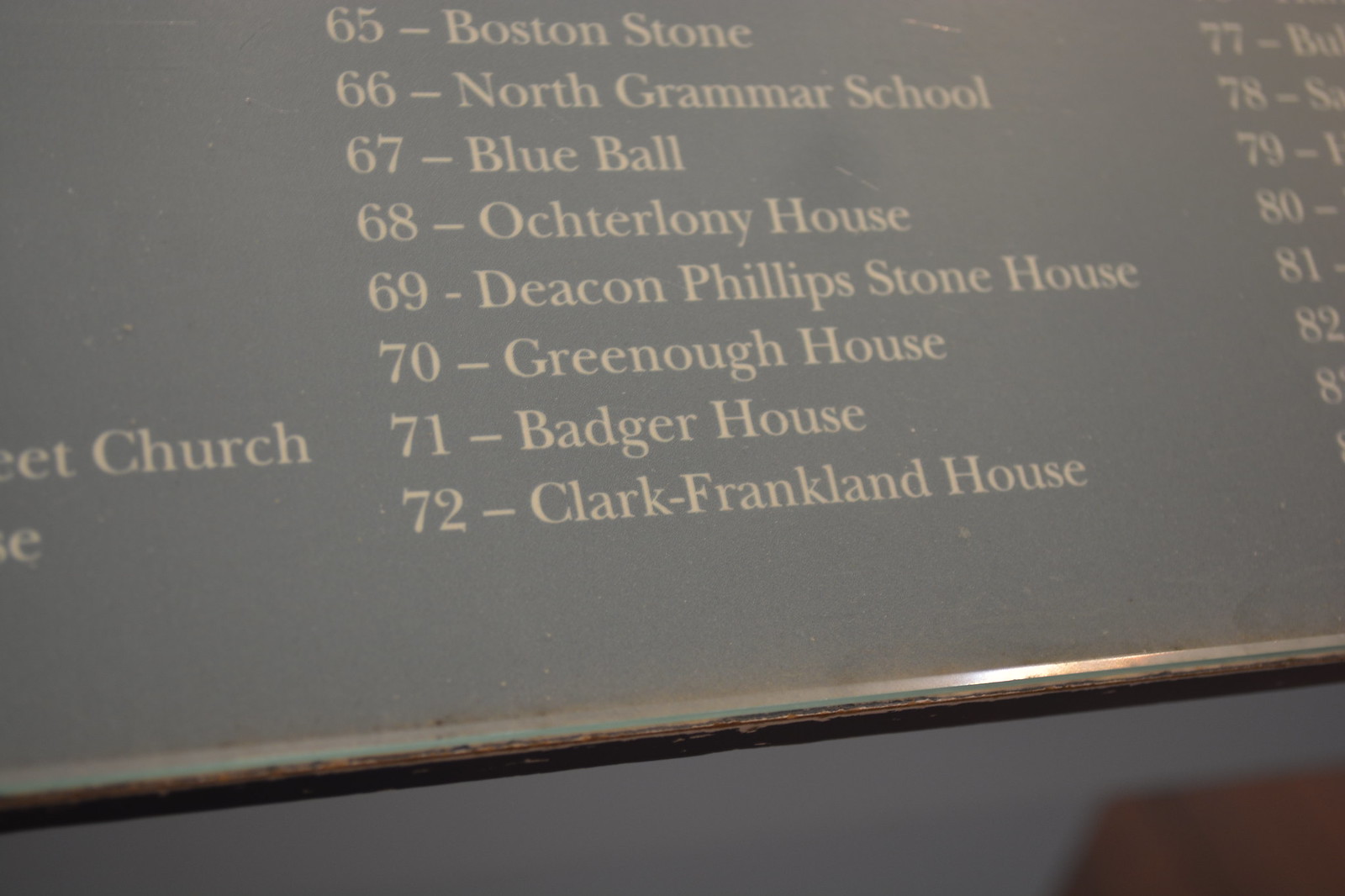This photograph features a close-up of a shiny, plaque-like directory with a dark brown border, appearing to be either indoors or outdoors, possibly at a monument. The plaque has a black or dark background with gold-colored lettering. Prominently displayed in the image are the lines of text listing a series of locations and their corresponding numbers: "65, Boston Stone; 66, North Grammar School; 67, Blue Ball; 68, Octorloney House; 69, Deacon Phillips Stone House; 70, Greeno House; 71, Badger House; 72, Clark Franklin House." On the left edge, the word "church" is partially visible, while the right edge shows partial numbers: "77, 78, 79, 80, 81, 82." The plaque takes up almost the entire frame of the image, and the colors visible include black, tan, brown, gold, silver, and white.